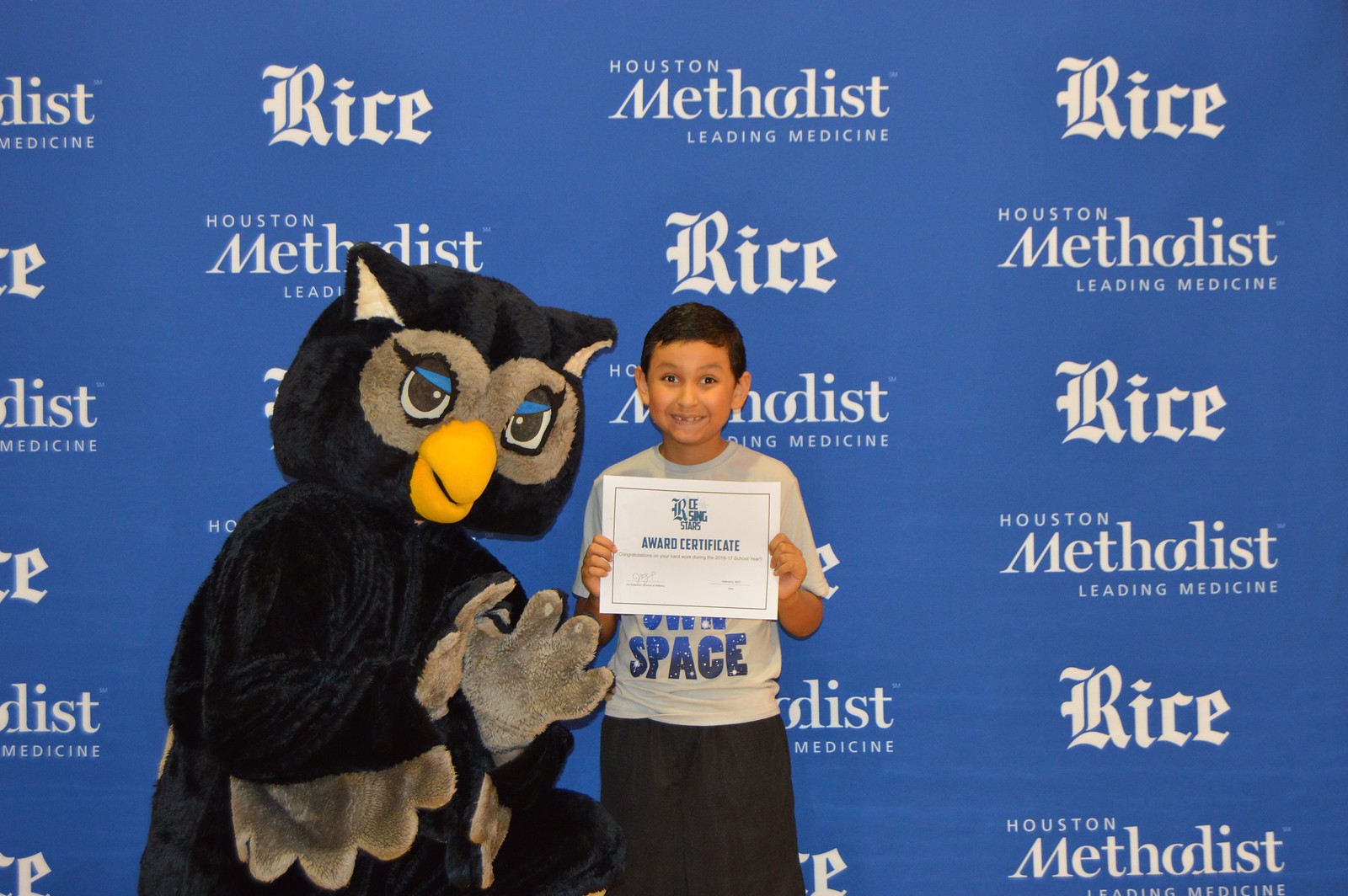In this color, landscape-oriented photograph, a young Latino-Hispanic boy around 10 years old is proudly holding up a white award certificate with blue lettering that reads "Rice Rising Stars Award Certificate," along with a signature on the bottom left corner. He is smiling at the camera, standing in the center of the image. The boy is dressed in black shorts and a gray t-shirt. To his right, on the left side of the image, is a mascot dressed as an owl, featuring predominantly black fur with gray on its palms, wings, and around its eyes, and a yellow beak. The owl mascot is crouched down, holding up its hands and waving. They are both posing in front of a dark blue banner that repetitively displays the words "Rice" and "Houston Methodist Leading Medicine" in white lettering. This scene captures a moment of celebration and achievement in a vividly detailed, representational realism style.